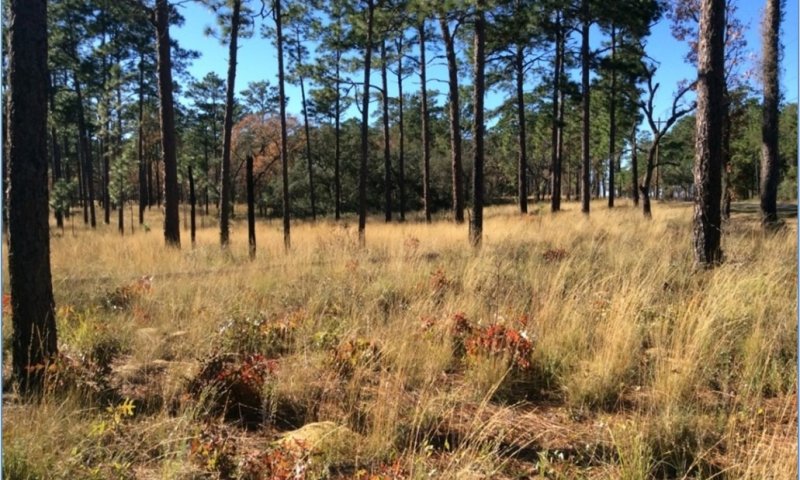The photograph captures a vast, slightly undulating grassy field dotted with sparse trees. The grass is predominantly long, dry, and yellowish-brown, interspersed with patches of light green and small red streaks, possibly from pine cones or dead plant matter. The trees are notably tall with thin, dark brown trunks, and their foliage is relatively sparse, showcasing hints of reddish-gold amidst the predominant green. This sparse arrangement gives way to a denser clustering of pines in the background, suggesting the field might be a clearing within a larger forest. The sky overhead is a vivid blue, providing a striking contrast to the earthy tones of the landscape below.